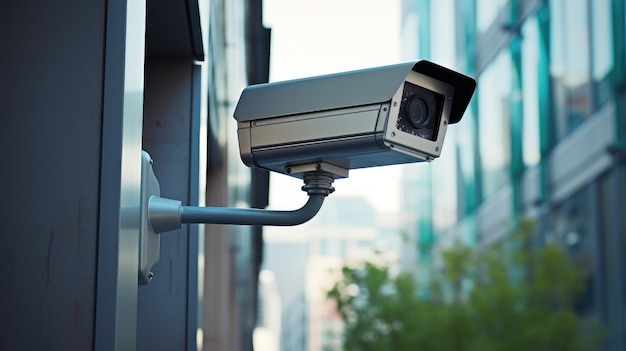The image captures a close-up, detailed view of a security camera mounted on the side of a modern building. The scene is set outdoors during daytime, with the sky and cityscape forming a blurred background. The camera, a rectangular prism made of stainless steel, features a small roof-like cover over its lens to protect it from rain and debris. The camera is affixed to a silver-colored metal arm extending from the left side of the image, which is part of the building’s exterior, also matching in silver or gray hue. In the far background, there are visible but unfocused elements like glass-clad office buildings and some greenery in the bottom right corner. The focus remains sharp on the camera, which is oriented slightly downward and angled towards the right side of the frame.